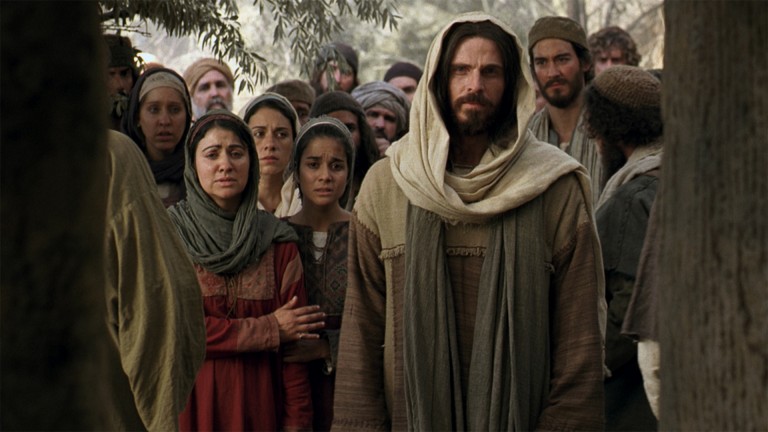In this scene from the TV show "The Chosen," we see a detailed and vivid depiction of Jesus of Nazareth surrounded by his followers. Jesus is centrally placed, wearing a greenish-brown robe with a dark green scarf and a white shawl around his head. His long, dark hair and beard are distinct features. He appears to be speaking or about to speak to the gathered group, who are attentively focused on him. The followers, both men and women, are dressed in traditional biblical attire with long robes and head coverings, predominantly in shades of brown, beige, and green. One woman in the background stands out in a red gown. The group is outdoors, standing under what seems to be an olive tree, with leaves hanging down, adding to the authentic historical atmosphere. The setting further suggests a scene rich with first-century cultural elements, emphasizing the show's effort to stay true to the period it portrays.